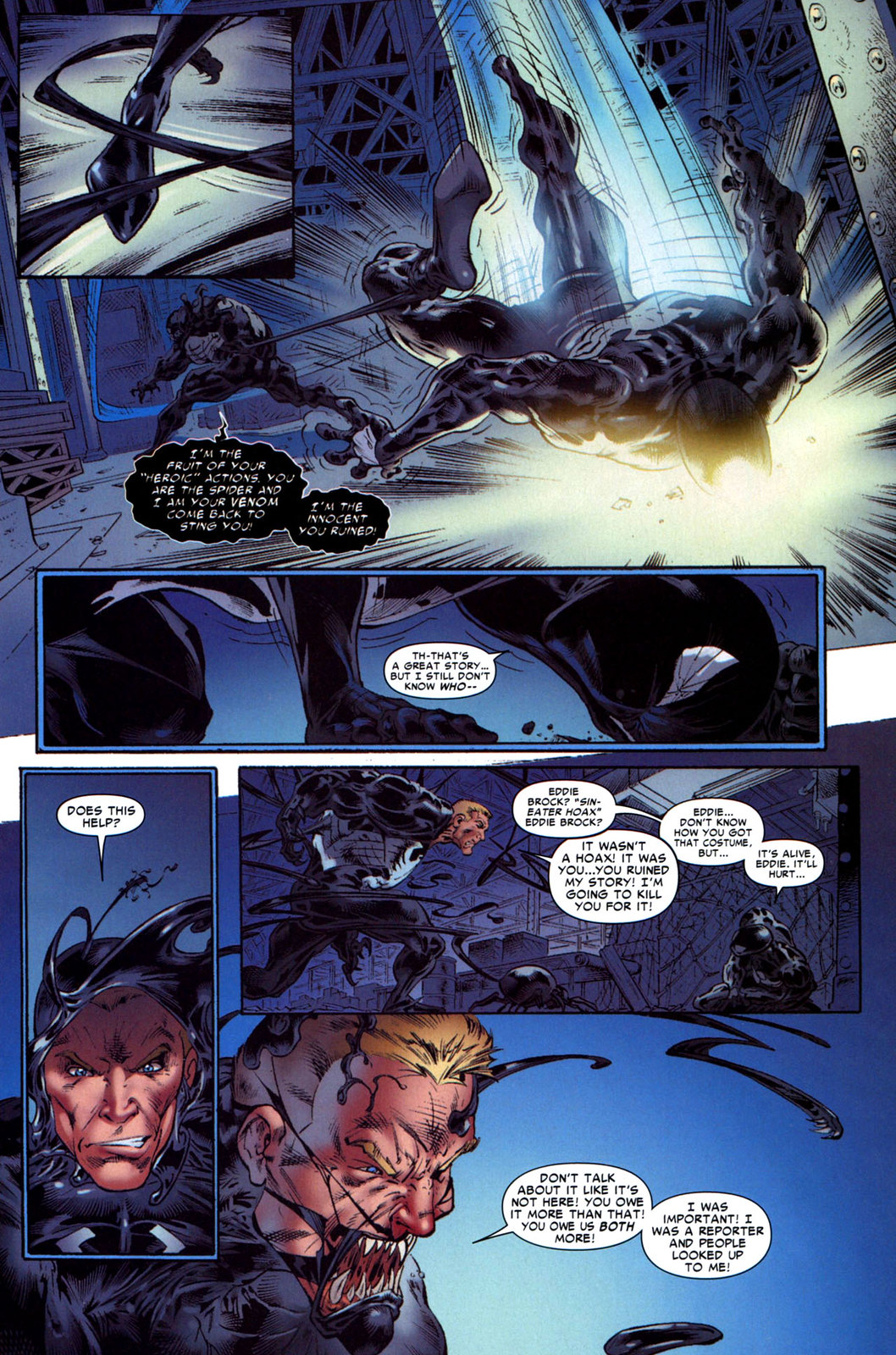This image is a detailed comic book page in portrait view, primarily using a blue and black color scheme. The upper left corner features a small square panel depicting a person's foot in a black, sock-like covering, with something wrapped around it, suggesting the person has been tripped. The action continues to the top third of the page, where you see a building in the background and a character falling headfirst, with another dark creature lunging at them and pulling on a string-like object.

Overlaying the main scene is a middle bar in landscape view, prominently showcasing the upside-down head of the falling character with a thought bubble stating, "That's a great story, but I still don't know who."

The bottom third is divided into three distinct images: the left panel is a close-up of a face saying, "Does this help?" The center panel depicts the same face, now revealing a man with short blonde hair and exaggerated vampire teeth, his wide mouth full of sharp fangs. The right panel shows a side view of this man with several thought bubbles emitting from him, the largest bubble containing the dialogue: "Don't talk about it like it's not here. You owe it more than that. You owe us both more. I was important. I was a reporter, and people looked up to me."

The overall background across these panels sways between dark blue and black, providing a dramatic and intense atmosphere to the comic.